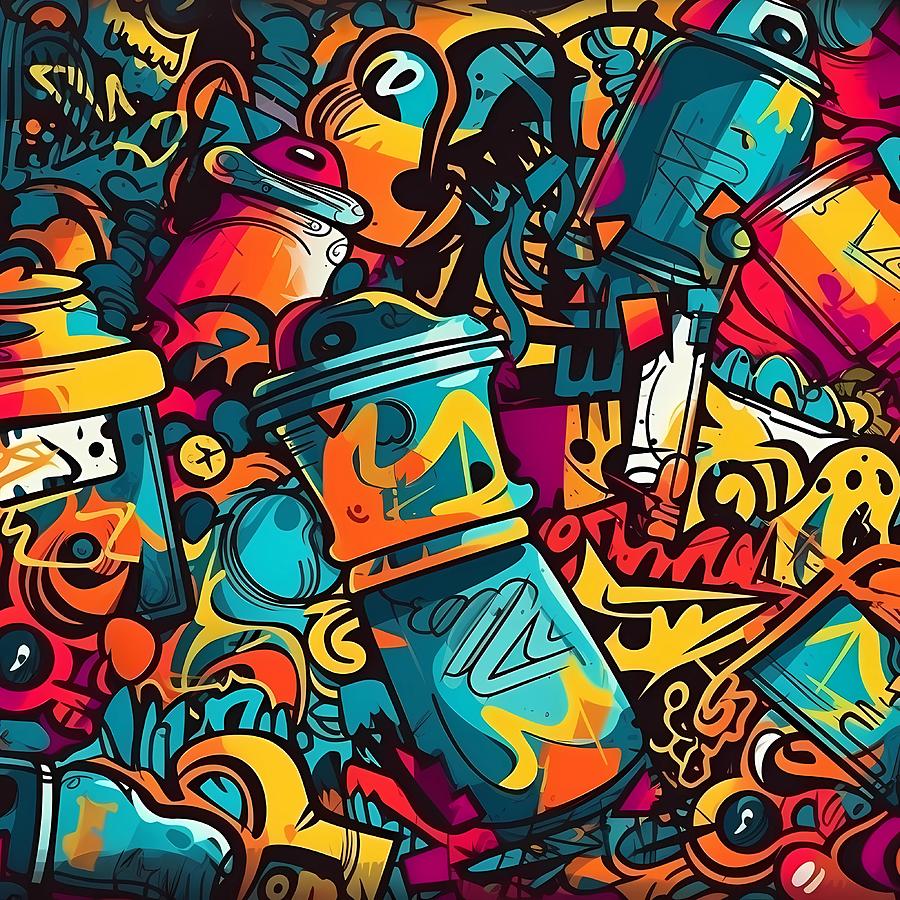This vibrant and colorful digital artwork, reminiscent of graffiti often found on urban walls, features an eclectic array of shapes and objects rendered in a cartoonish style. The square-shaped image is dominated by a chaotic mix of blue, yellow, orange, pink, and red hues, with accents of black and white. Prominently, a blue, almost cylindrical object with yellow and orange lines draws the eye, alongside what appears to be a bottle-like figure in shades of pink and orange. The artwork is devoid of any recognizable text, emphasizing abstract forms that evoke the appearance of spray cans, cups, and possibly chess pieces, scattered randomly across the canvas. The top left-hand corner is particularly blue with yellow squiggles, whereas the bottom right bursts with red hues. Despite the lack of repeating patterns, the vibrant, clear, and vibrant cartoon-like shapes unify the piece, bathed in bright, natural lighting which highlights its dazzling colors.